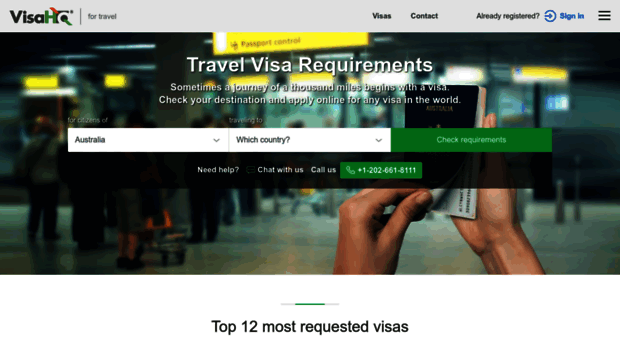### Detailed Descriptive Caption for the Image

This image is a screenshot of a website's homepage with an intricate and well-organized layout designed for ease of navigation. At the very top, there is a light gray header spanning the width of the page. On the left side of this header, "VISA" is inscribed in gray text. 

Adjacent to this, slightly to the right, is an "HQ" icon. The "H" within the icon is green, while the "Q" is stylized, featuring an orange line ascending to the left at a 45-degree angle and a green line descending to the right at the same angle. Bridging this section and the next is a medium-gray vertical separator line.

Centrally positioned in this header section sits more gray text, reading "FOR TRAVEL." Following a segment of negative space, the header continues to list options in gray text: "VISAS," "CONTACT," followed by another patch of negative space, and then "ALREADY REGISTERED!" 

To the far right, there is a blue circular icon encompassing a rightward-pointing blue arrow. Accompanying this icon is "SIGN IN" rendered in blue text, followed by a gray hamburger menu icon positioned at the extreme right end of the header.

Below this header, a blurred backdrop photograph reveals what appears to be an airport security line, bathed in blue and gray hues. Central to this photograph are two hands holding up a blue passport adorned with a golden emblem.

Overlaying the image is prominently styled white text, centered near the top, stating "TRAVEL VISA REQUIREMENTS." Directly below in smaller white text are the lines: "SOMETIMES A JOURNEY OF A THOUSAND MILES BEGINS WITH A VISA. Check your destination and apply online for any visa in the world." 

Beneath this textual overlay lies a series of drop-down menus set against white backgrounds, facilitating user interaction. Positioned to the right of these drop-down menus is a green button with white text that reads "CHECK REQUIREMENTS."